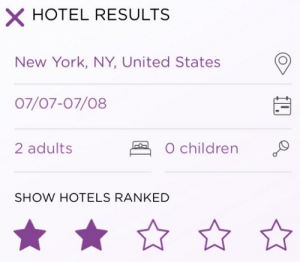The image depicts a screenshot of hotel search results. It showcases a small interface with a light gray background. In the top left corner, a purple 'X' icon is followed by the bold, black, capitalized text "HOTEL RESULTS." Below, in purple text, it specifies the location as "New York, New York, United States." To the right of this is a BAP icon button indicating the user's current location.

Further down, the date range "00/00 to 07/08" is displayed in purple, accompanied by a gray calendar icon on its right. The search criteria specify "2 Adults," illustrated with a gray bed icon, and "0 Children," indicated by a gray rattle icon. These details are highlighted in purple text.

At the bottom, the descriptive text reads "SHOW HOTELS RANKED" in dark, bold, capital letters. Adjacent to this text are five star icons, the first two are fully filled in purple, while the remaining three stars are outlined in purple but remain unfilled.